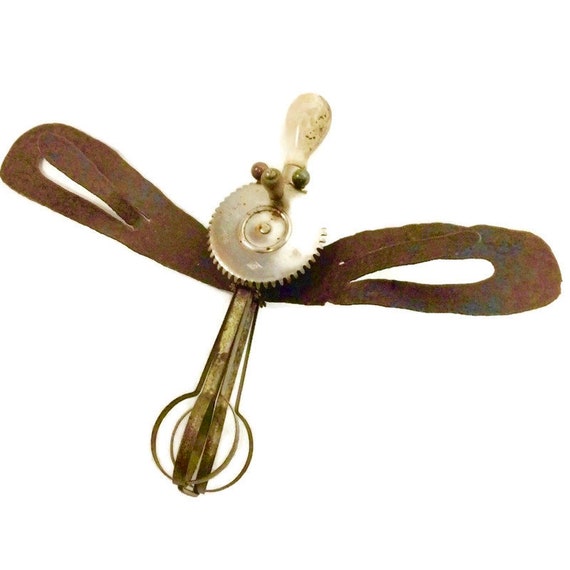This color photograph, taken in landscape orientation, showcases a vintage handheld kitchen beater artfully presented against a stark white background, lending a floating appearance to the device. The top of the beater features an elliptical, whitish handle, possibly made of plastic or marble, that tilts slightly to the right. Below the handle is a striking silver mechanism with intricate gears and teeth, adorned with three small balls in green, reddish, and gray hues.

The lower section of the beater comprises three brass-colored whisks that intersect and point in various directions, forming a characteristic antique design. Beneath this gleaming silver apparatus lies a brown leather strap gathered at the center, suggesting it could be a mask-like adornment to the beater, covering the area that would traditionally align with the bridge of one's nose and around the eyes. The harmonious blend of materials and colors, alongside the photo’s realism, brings out the rich, textural details of this historical kitchen tool.